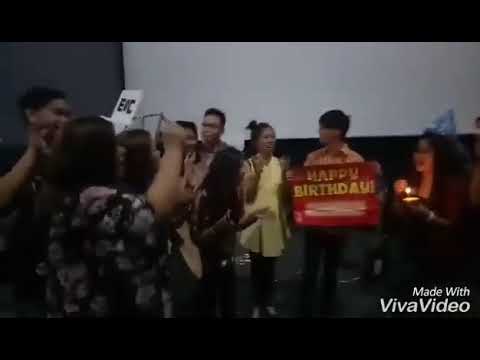This image depicts a celebratory scene with a group of eight people, apparently of Asian descent, standing in what appears to be a large room. The group's formation consists of a row of five individuals, with two more standing closer to the camera on the left. The overall image quality is poor, marked by blurriness and blocky resolution.

In the back row, starting from the right, there is a man in a pink shirt holding a large red sign with yellow text that reads "Happy Birthday." The sign’s lower section is indiscernible, likely due to the image’s blurriness. To his right is a shorter woman holding a candle in her hand, wearing a blue birthday cap. To the left of the man, there is a woman dressed in a yellow dress, followed by a man who appears to be wearing glasses, though the details are unclear. Next to this man, there is either another woman or possibly a child, obscured and hard to distinguish due to other people partially covering them.

In the front left, a taller man is captured clapping, adding to the celebratory atmosphere. Closest to the camera, on the left side, is a woman with her back turned, her right arm raised in a gesture resembling a fist bump. She is dressed in a black dress adorned with white flowers.

The photograph is overlayed with thin black bars at the top and bottom. In the lower right corner of the image, white text reveals it was "Made with Viva Video."